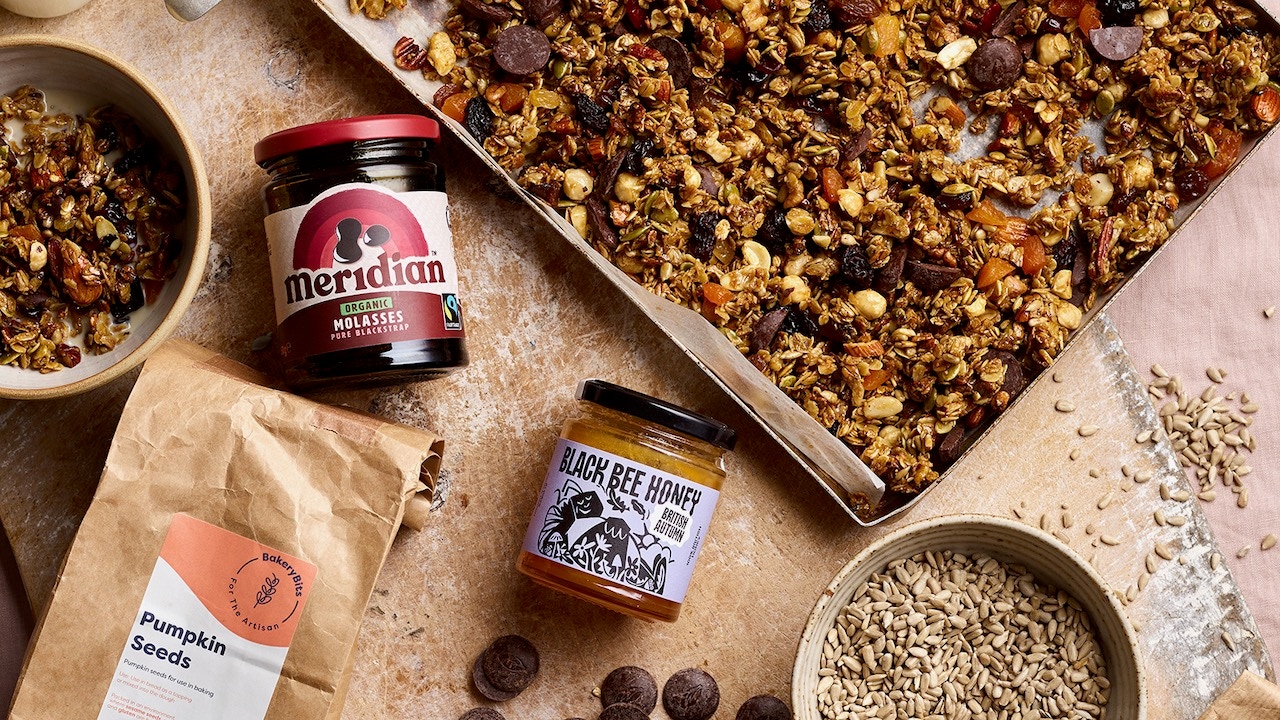The image depicts a rectangular photograph, approximately six inches wide and four inches high, showcasing a variety of items arranged on a crackled brown and white countertop. Dominating the scene is a large, rectangular metal tray lined with wax paper, filled with an assorted granola mix. The granola features a colorful array of oats, chocolate chips, almonds, raisins, pumpkin seeds, and pieces of dried fruit, creating a contrasting tapestry of browns, yellows, purples, and orange hues. 

Adjacent to the tray, we see two jars. The first jar, positioned in the foreground, is labeled "Meridian Organic Molasses" and features a red cap, containing a dark, viscous substance. To its right is another glass jar labeled "Black Bee Honey" with a black lid and a purple label, filled with amber-colored honey. 

On the left side of the image, a brown paper bag with a dual-colored label that reads "Pumpkin Seeds" can be seen. Above this bag is a bowl containing the same granola mix found on the tray. 

Additionally, in the lower right-hand corner, there is another bowl, partially visible, containing small seeds that appear to be either sesame or sunflower seeds. The overall scene suggests the preparation or serving of a homemade granola mix on a kitchen countertop.